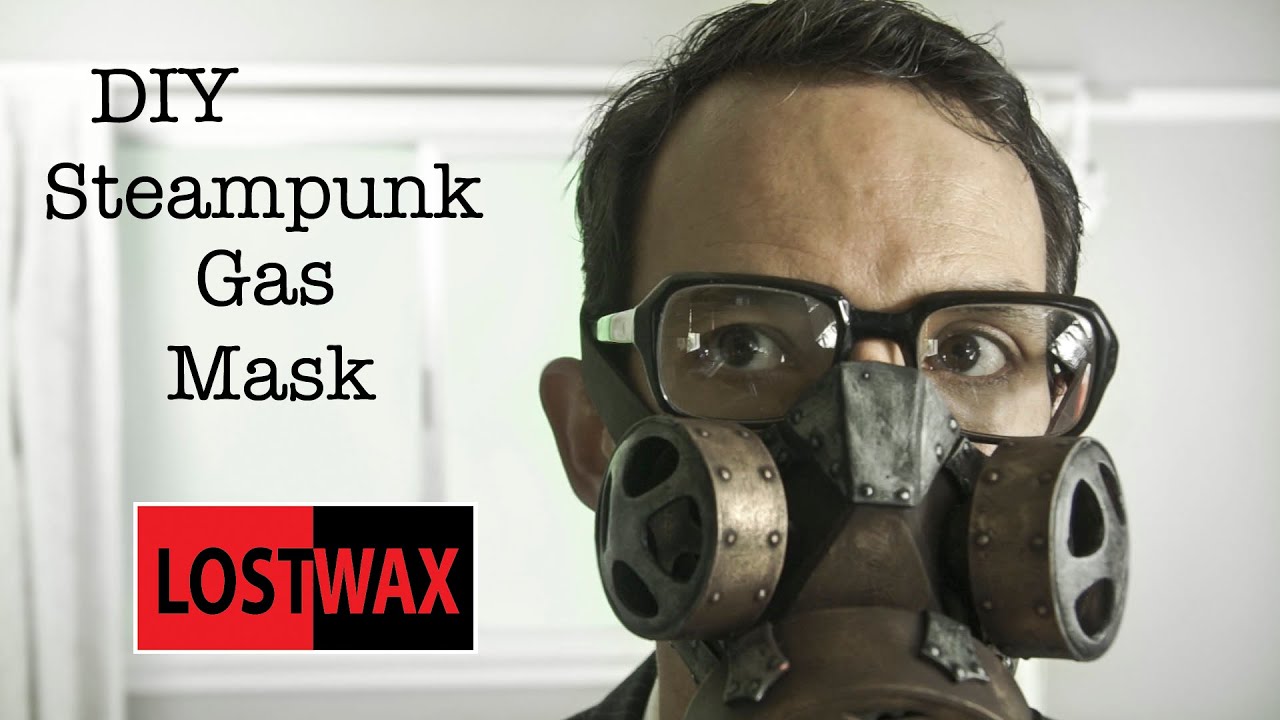This advertisement showcases a DIY Steampunk Gas Mask prominently. The black text for this title is positioned in the upper left section of the image. Below it, there's a distinctive logo for "Lost Wax," a wide rectangular design split into two parts: "Lost" in black text on a red background, and "Wax" in red text on a black background. The central figure in the close-up image is a white man with short brown hair, wearing very thick black-framed glasses. The elaborate gas mask he wears has a distressed, rusted iron appearance with ornate, riveted metal-like pieces enhancing its traditional design. The mask, covering his nose, mouth, and cheeks, gives a steampunk aesthetic, perfect for enthusiasts of this genre. The background includes muted, slightly blurred elements like a window and curtains, and overall, the image is set against a white backdrop for clarity. This detailed representation not only highlights the mask's intricate design but also situates it in a steampunk context, making it a unique costume accessory.